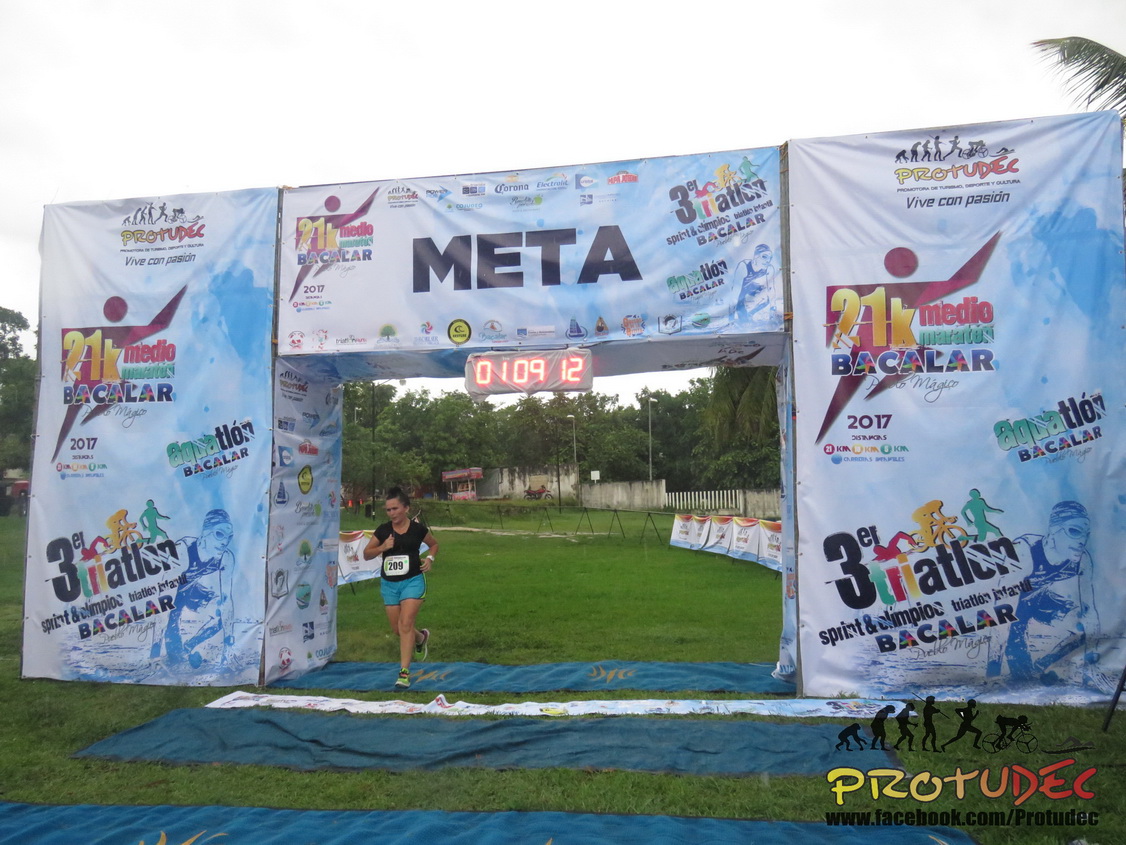This captivating photograph captures the finish line of a race, possibly a triathlon, set outdoors on an overcast day. A woman with her dark hair pinned up, dressed in a black short-sleeve shirt, sky blue shorts, and bright green running shoes, is captured just past the finish line. Pinned to her waist is the number 209, printed in black on a white background. Her time, displayed in red digital numbers, reads 01:09:12. The finish line is marked by a squared-off white canvas arch adorned with various advertisements, including the prominent word "META" in large black letters, and references to a 21K race and triathlon. In the background, the lush green grass contrasts with the overcast sky and the occasional palm tree, creating a striking outdoor scene. On the lower right corner of the arch, there is a web address: www.facebook.com/pro2deck. The clear and peaceful atmosphere of the finish line is accentuated by the absence of other participants or onlookers in the immediate vicinity.